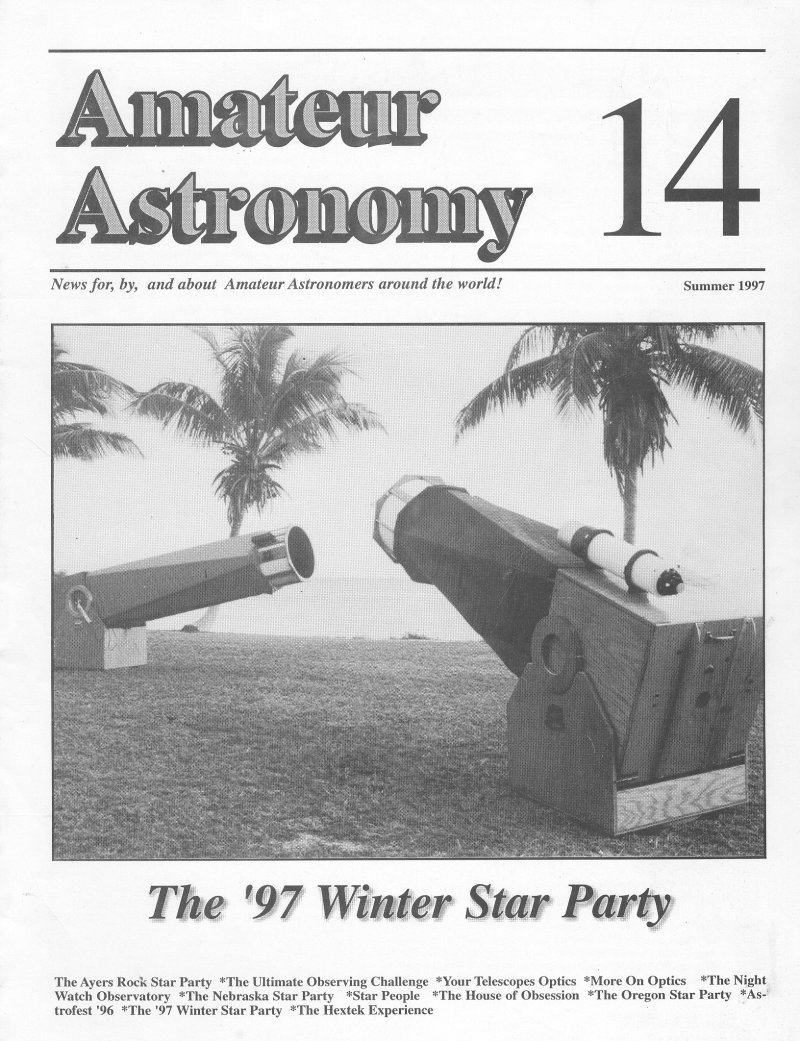The image showcases the cover of "Amateur Astronomy," issue number 14, dating back to the summer of 1997. Rendered in a faded black and white, the magazine cover prominently features the headline "News for, by, and about amateur astronomers around the world!" Near the top right corner, the issue number "14" and the date "Summer 1997" can be clearly seen. Central to the cover is a monochrome photograph of two enormous telescopes positioned on a grassy lawn. These telescopes are directed slightly upward and point towards each other, framed by palm trees in the background, hinting at a beachside location. Beneath the image, the headline "The 97 Winter Star Party" is boldly displayed, followed by a list of article titles in smaller text, including "The Irish Rock Star Party," "The Iron Observing Challenge," "Your Telescopic Optics," "More on Optics," "The Night Watch Observatory," "The Nebraska Star Party," "Star People," "The Home of Obsession," "The Oregon Star Party," "05," "The 1992 Winter Star Party," and "The Heslick Experience." The serene and clear sky in the backdrop suggests ideal conditions for stargazing during this star party event.